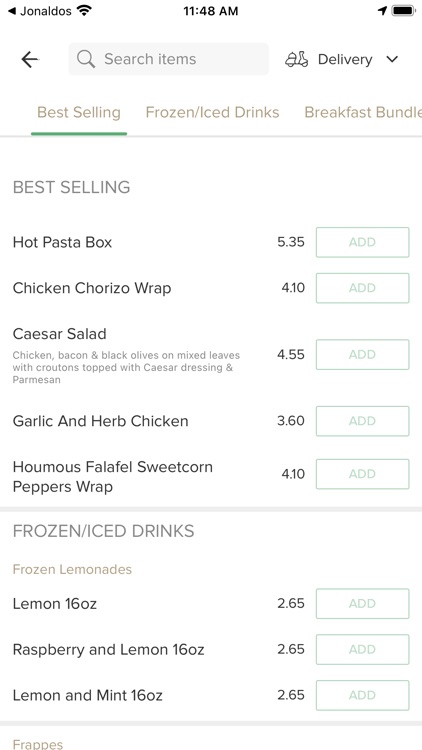The image is a color, portrait-format screenshot of a smartphone display connected to the Jonaldos network, evidenced by the network name and full signal bars shown in the top left corner. The time indicated is 11:48 a.m., and a 'delivery' icon is featured on the top right.

The app interface displays various food and drink tabs including "Best Selling," "Frozen Ice Drinks," and "Breakfast Bundle," with the user currently browsing the "Best Selling" tab. This section lists several popular food items available for purchase:

- Hot Pasta Box: $5.35
- Chicken Chorizo Wrap: $4.10
- Caesar Salad: $4.55
- Garlic and Herb Chicken: $3.60
- Hummus Falafel Sweet Corn Peppers Wrap: $4.10

Each item displays an "Add" button for easy inclusion into a cart for streamlined purchasing. Additionally, the "Frozen Ice Drinks" section mentions options like an "11, 16-ounce" drink, among others. The currency is unspecified, but the prices suggest a detailed menu for convenient ordering.